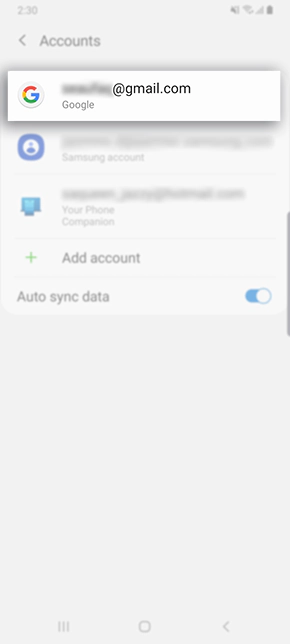A screenshot of a cell phone's account settings interface. The background is gray, with a blurry overlay effect on the entire screen. In the upper left-hand corner, the time is displayed. On the right side, there are icons for battery, signal reception, and Wi-Fi status. 

Two lines down from the top left, there is a left-pointing arrow icon shaped like a sideways "V". About five spaces to the right in larger font, the word "Accounts" is displayed. Beneath this, there is a prominent white rectangle with black shading around its edges. Inside this rectangle, on the left, is the Google "G" logo encircled by a light gray outline. Next to the logo is a partially blurred Gmail address, showing only the "@gmail.com" domain clearly, with "Google" written below it.

Below this section, there are two icons, but the labels or images to the right of these icons are blurred out, making them unreadable. Underneath these icons is a green plus sign followed by the text "Add account." At the bottom, there is an option labeled "Auto-sync data" with a toggle switch on the right. The toggle switch is turned on, indicated by its aqua blue and white color.